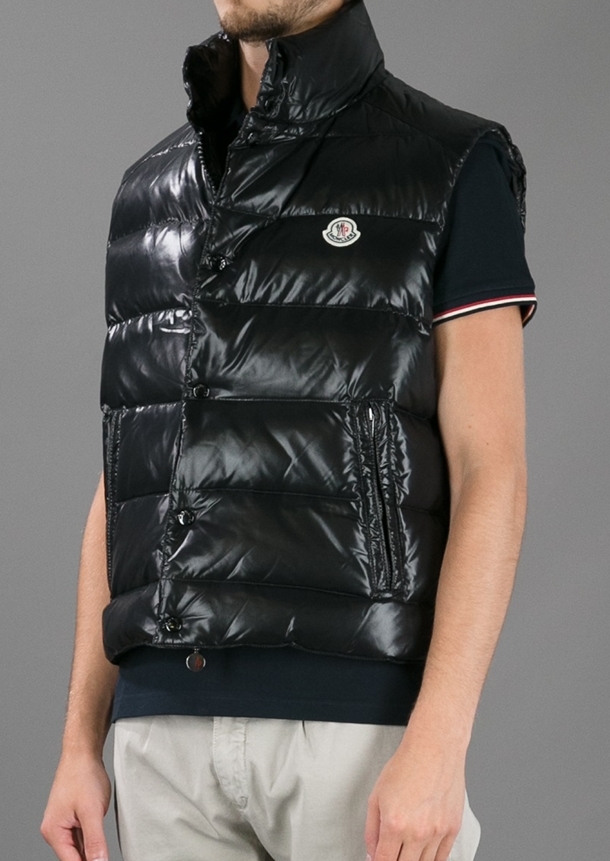In this detailed photograph, a man, whose face is mostly cropped out showing only his chin with a hint of a small beard and five o'clock shadow, is wearing a sleek, shiny black puffer vest, which features a distinctive bubble design. The vest is sleeveless and has a high collar, with a barely readable small white emblem on the left chest that's round in shape. The vest's material seems to have a leather-like sheen. Underneath, he's wearing a black short-sleeve t-shirt, adorned with red, white, and black stripes around the sleeves. His lower attire consists of khaki pants. The image primarily showcases his upper body with his arms held at his sides, and the background is a plain gray.